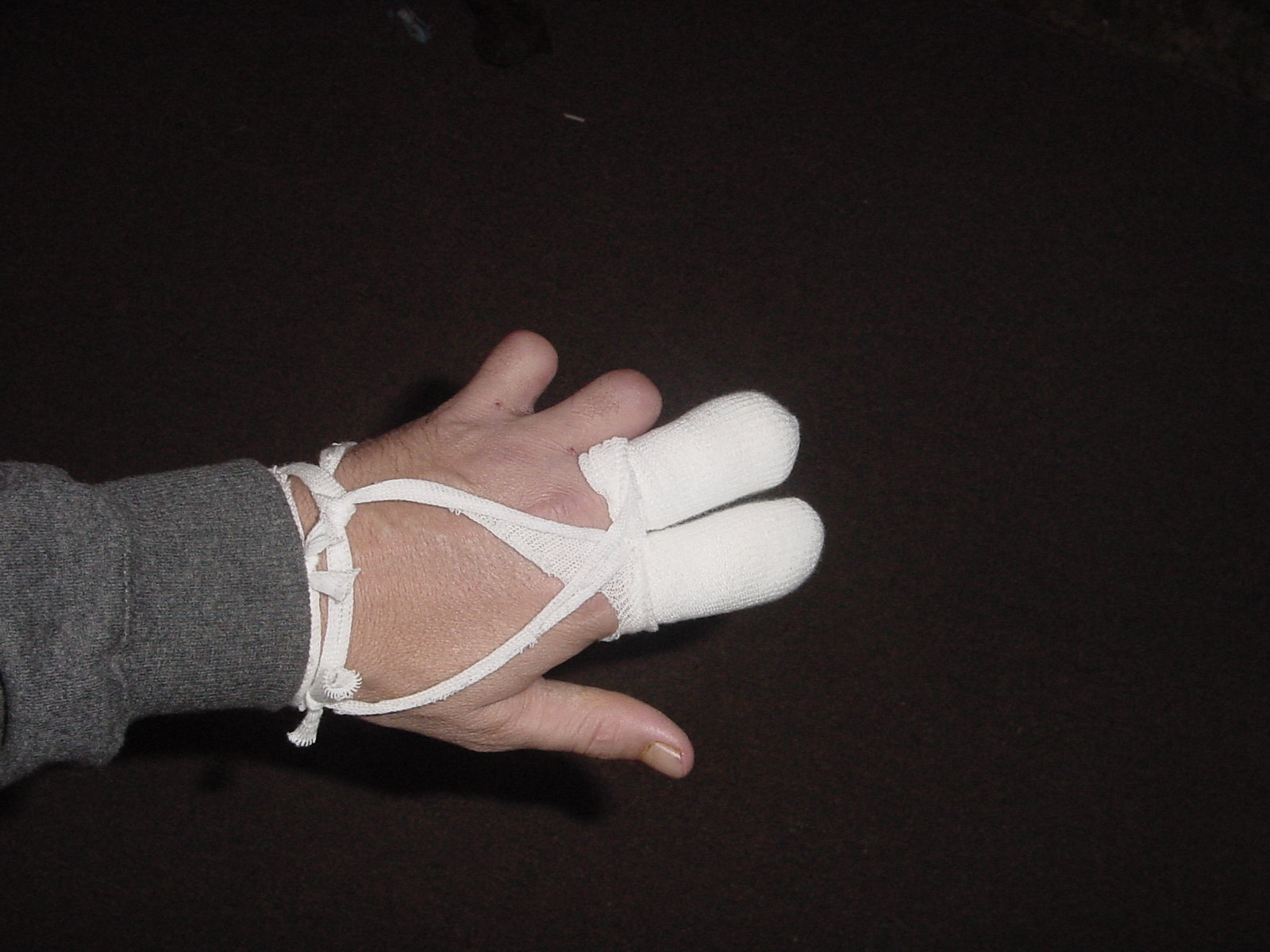The image is a color photograph with a completely black background. It showcases a person’s left hand coming in from the bottom left corner of the photo. The arm is clad in a dark gray knit sweatshirt, featuring a ribbed fabric at the wrist. The hand is depicted in full, revealing that the top halves of the pinky and ring fingers are missing. The middle and index fingers are heavily wrapped in thick white bandages resembling gauze wraps, which extend down in strands to wrap around the wrist. The thumb appears uninjured and normal. The identity of the individual, including their gender, is not discernible from the photograph. The overall impression is of a person who has recently lost parts of two fingers and is in the process of healing with the help of substantial bandaging.